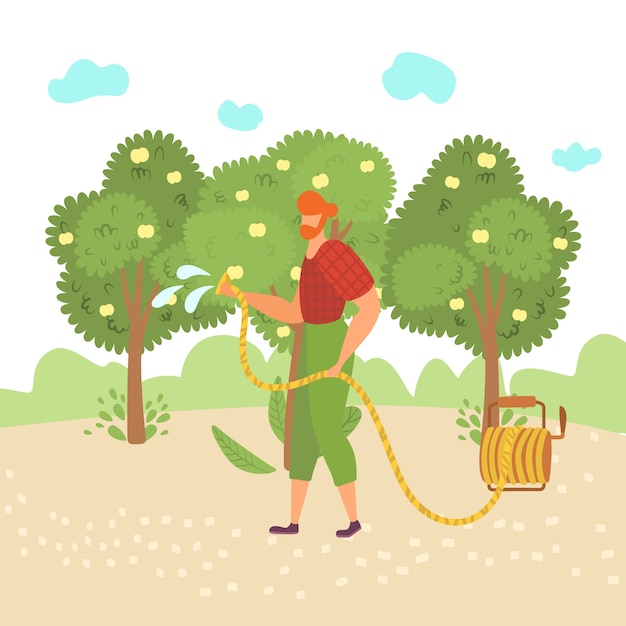In this simplistic, corporate-style cartoon image, we see a red-bearded man with a matching pompadour, dressed in a red checkered shirt and green pants, watering the landscape with a yellow, striped, retractable water hose mounted on a brown rolling device. The character, notable for his lack of facial features apart from his distinctive hair, stands out against a background that includes light blue clouds in a white sky, three green trees bearing white fruit, and lighter green shrubs. The ground appears beige with a hint of a pathway marked by white polka dots, while the overall color palette is rich with greens and browns, giving the scene a simplistic yet colorful charm.